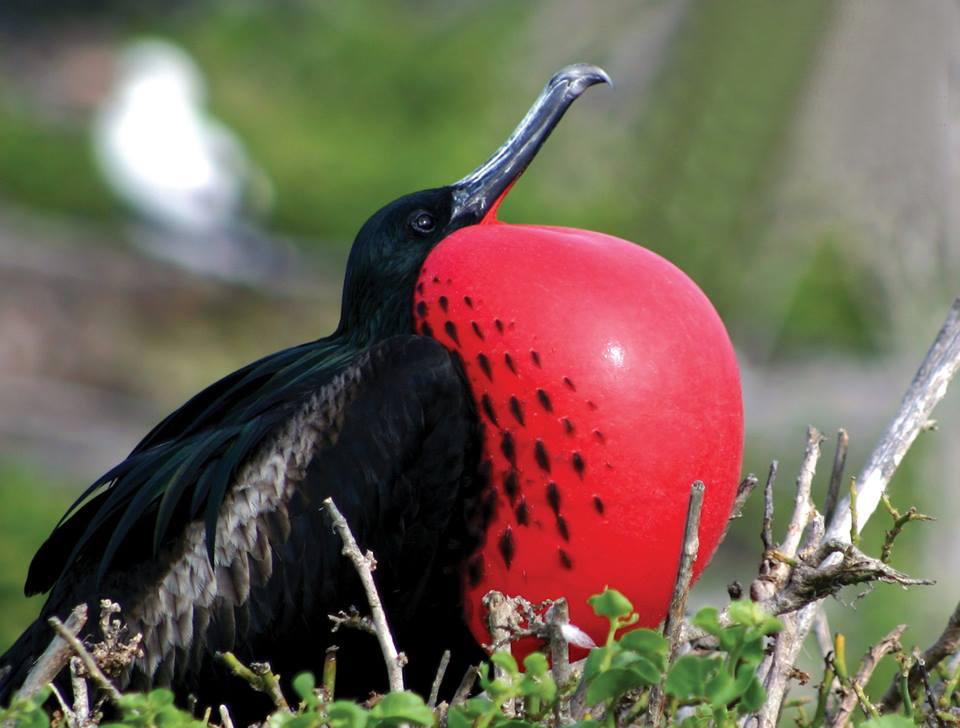This nature photograph captures a close-up of a striking black bird in the midst of a display. The bird, perched on a branch adorned with small green leaves and broken sticks, has a predominantly black body with some patches of white feathers and brown. Its most prominent feature is a vibrant, bright red throat that is hugely puffed out, resembling a balloon or half an apple, with small black dots speckled across it. This dramatic inflation, likely part of a mating call or display, is vividly contrasted against the bird’s elongated grayish beak, which tapers into a slight downward curve at the tip. The blurred background, a mixture of green and gray hues, keeps the viewer’s attention firmly on the bird and its eye-catching, swollen throat. With no other birds in sight, this solitary creature seems intent on attracting a mate or making a vocal proclamation in its lush, verdant surroundings.